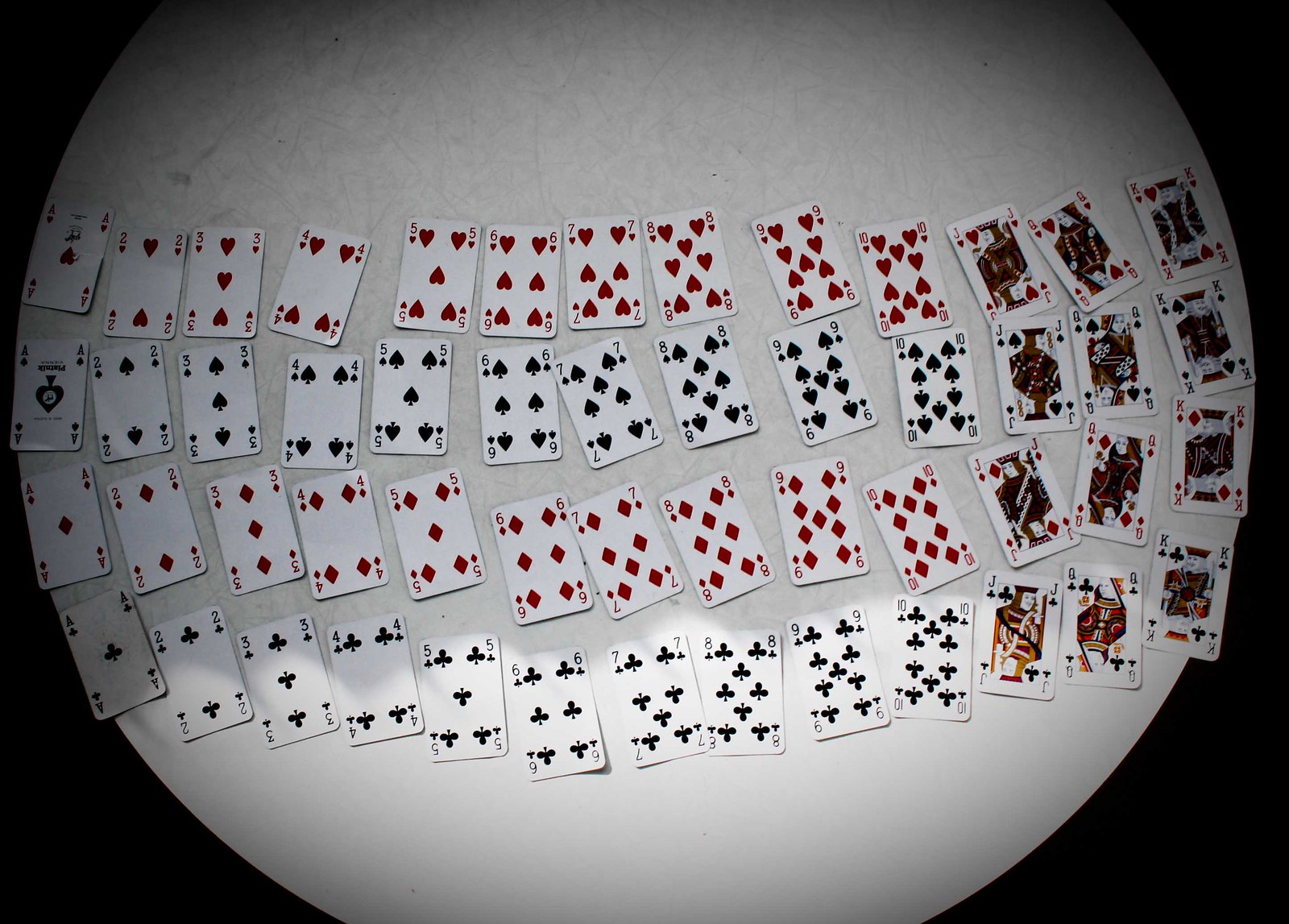The image depicts a meticulously arranged spread of playing cards on a pristine white surface. The photograph has rounded edges with a black border, accentuating the slightly three-dimensional appearance of the circular white background. The cards are laid out horizontally in four rows, each row slanted slightly off-center rather than perfectly straight. This creates a visually dynamic arrangement.

Starting from the top, the first row consists entirely of red cards, the second row of black cards, the third row of red cards again, and the fourth row of black cards. The cards are organized by suite, progressing sequentially from hearts to diamonds in the red rows, and from clubs to spades in the black rows. Each card is face up, showcasing a full set from ace through king. The cards themselves are in immaculate condition, appearing crisp and new, lacking any signs of wear or aging. The arrangement does not suggest any particular card game in progress, but rather, presents a visually pleasing display of alternating colors and orderly sequences.